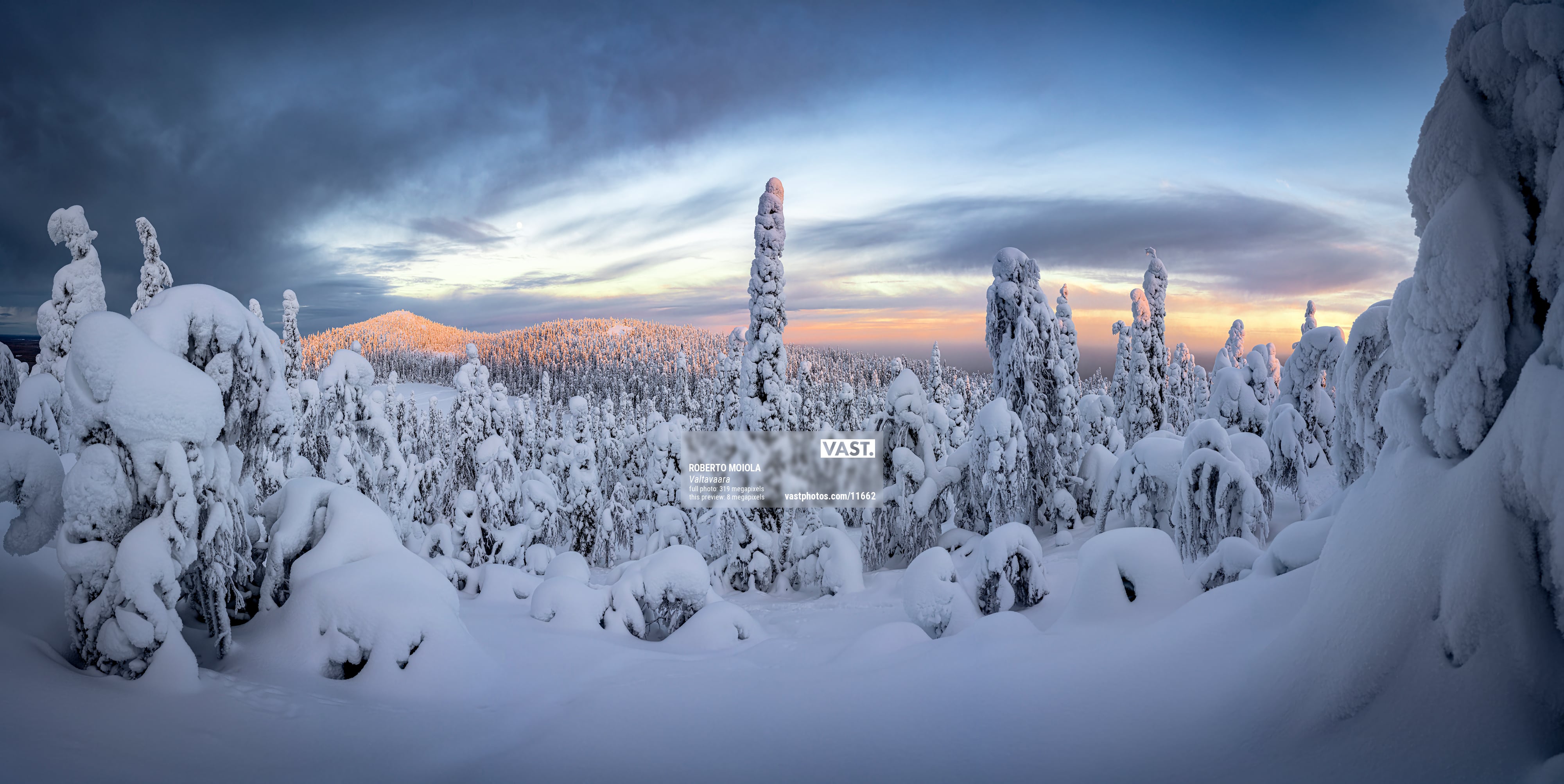The photograph, taken outdoors, captures a snow-covered mountainous landscape at sunrise. Tall, thin trees stand in the deep snow, their branches heavy with the white blanket. In the background, hilltops are bathed in a golden hue from the rising sun, while the rest of the scene remains in cool, blue-toned shadows. The sky features a dramatic gradient, with dark clouds on the left, transitioning to lighter blues and yellows near the horizon, and blending into darker blues at the top. A watermark is centered within the image, subtly marking the serene, natural beauty depicted.